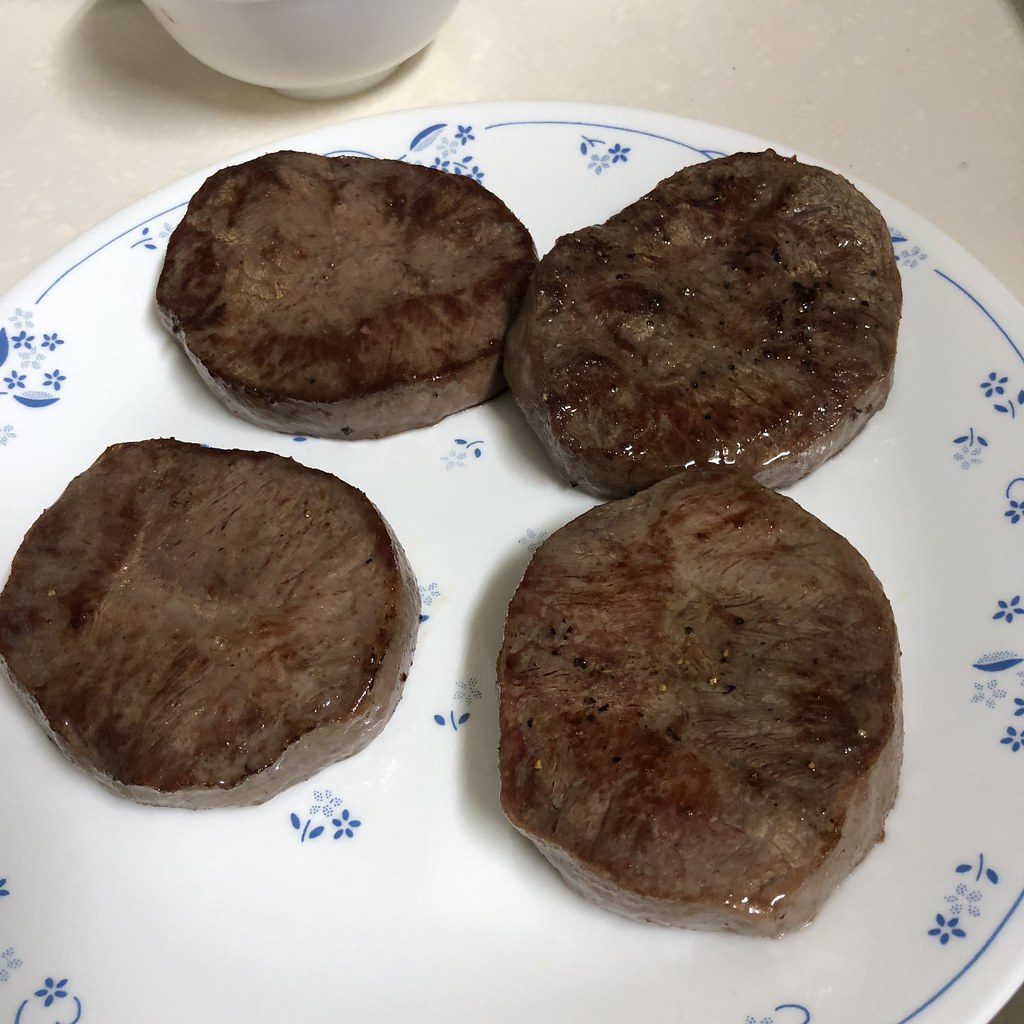In a cozy kitchen setting, the photograph captures a white plate adorned with small blue flowers and a blue trim along the edge, resting on a white counter. The focus of the image is on four freshly cooked breakfast sausage patties arranged almost in a circular pattern with two at the top and two at the middle of the plate. The sausages, approximately half an inch thick, exhibit a brownish-gray hue with seared char marks and glistening with shiny grease, indicating they haven’t been patted dry yet. Light sprinkles of pepper can be seen on the sausages, adding texture to their surface. Towards the upper left side of the image, the base of a white coffee cup is partially visible but cut off, while the background remains a clean white, emphasizing the simplicity and freshness of the meal.